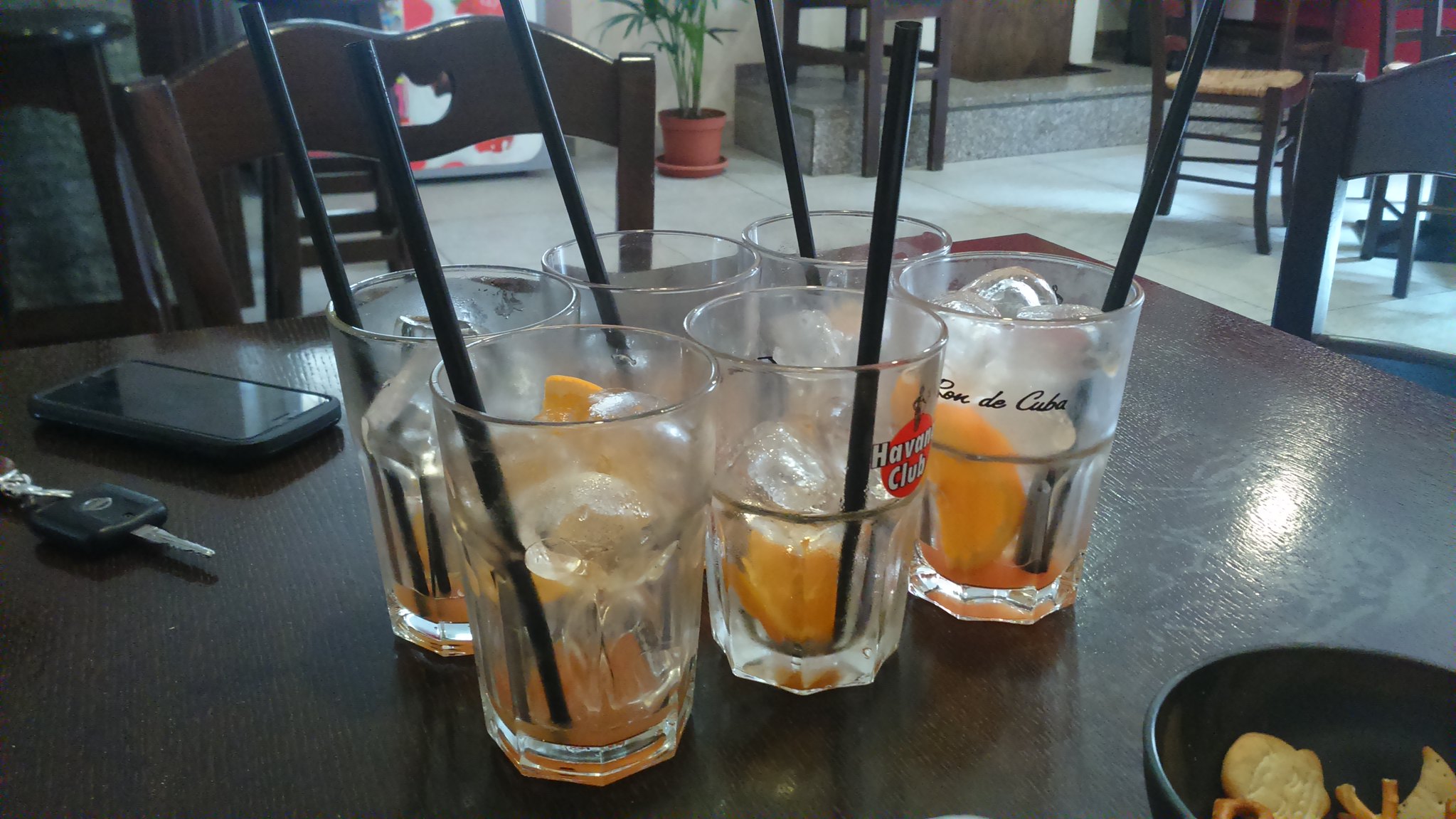The photo depicts the interior of a Cuban restaurant featuring a dark brown wooden table surrounded by matching dark brown wooden chairs. The table prominently displays six clear glass cups, each containing a considerable amount of ice cubes and slices of citrus fruit, including oranges and lemons. Each glass is equipped with a black straw, and one glass bears a red emblem with the words "Havana Club," while another has cursive black lettering stating "Ronde, Cuba." On the table, there's also a small, dark-colored bowl filled with pretzels and face-shaped crackers. Additionally, a black smartphone with a shiny glass screen and a black square car key with a silver key attached lie on the table. The floor consists of light tan or white tiles, and the walls of the restaurant are a tan color. In the background, more tables and chairs are visible, as well as what appears to be a vending machine and a step leading, possibly, to the restrooms.